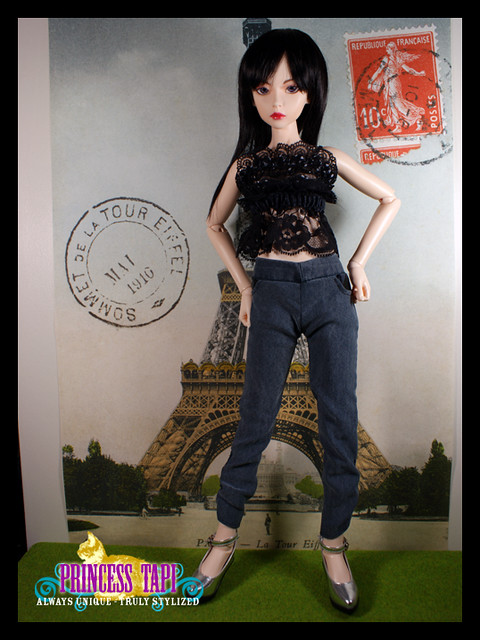This detailed image features a fashion doll with dark hair, striking a confident pose with her hands on her hips. She is elegantly dressed in a lacy black blouse, dark slacks, and silver high-heeled shoes. The doll is situated on a green surface that resembles grass. Behind her, there is a postcard of the Eiffel Tower, prominently postmarked "Sommet de la Tour de Fels, May 1910" on the left side. The upper right-hand corner of the postcard features a red, partially torn postage stamp with a postmark over it. The entire setup appears to be a meticulously staged photograph, well-lit to prevent any distracting shadows. The image is enclosed by a black border and bears the logo of Princess TAPP, who promise their dolls are "Always unique, truly stylized," displayed in the lower left corner.